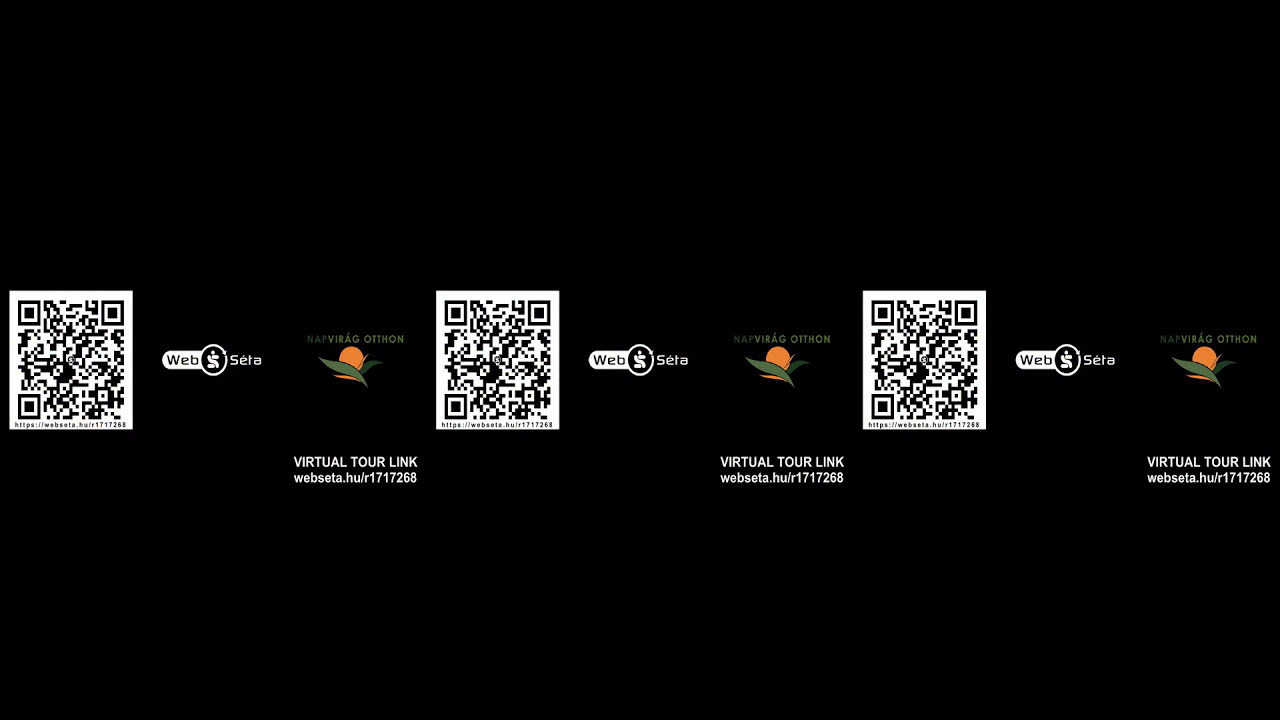The image features a black background divided into an upper, middle, and lower third. The upper and lower thirds are completely black, providing a stark contrast to the central part of the image. Occupying the middle section, there are three QR codes, each depicted as white squares with intricate black patterns. At the center top of each QR code is a black square within a white square encased by another black square. 

Between each QR code, the text "Virtual Tour Link" is prominently displayed, followed by the URL "webceta.hu/r1717268." This set of text appears three times beneath each respective QR code. To the immediate right of the central QR code and at the left edge, there is a logo comprising an orange with green leaves, accompanied by the text "Webceta." This logo is placed at the right mid-center and left mid-center respectively. The words "Virtual Tour Link" and the URL are repeated consistently to provide clarity. 

Overall, the design is clean and professional, facilitating easy scanning of the QR codes and quick identification of the essential information.